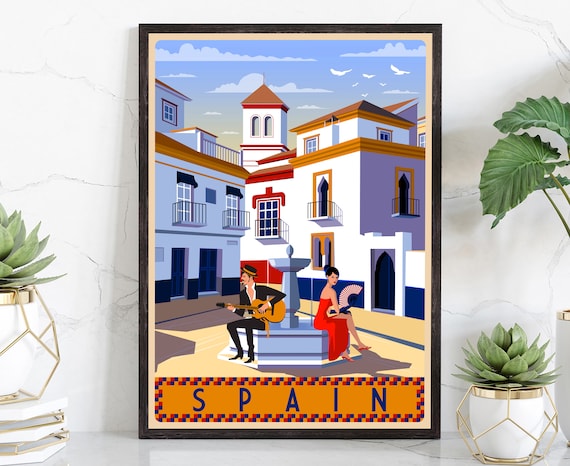The image depicts a framed, cartoon-like drawing representing Spain, leaning against a weathered, white plaster wall covered in delicate, eggshell-like cracks. The artwork showcases a tranquil scene set around a concrete fountain, with two central figures: a man on the left, in a black hat, black boots, and an unbuttoned shirt, strumming a guitar; and a woman on the right perched elegantly, dressed in a strapless red dress and red high heels, fanning herself with a spiraled red fan. Her hair is styled in a bun, giving her a poised appearance suitable for a formal dance. The backdrop features white stone buildings with balconies typical of Spanish or European architecture, and a prominent red steeple or bell tower at the center. The sky transitions from yellow to blue, suggestive of a sunset, and is scattered with white birds. Below the figures, the word "Spain" is spelled out in blue, widely-spaced letters against a yellow ground. The painting is bordered by a pattern of alternating blue, yellow, and red squares, all enclosed within a gray frame. Flanking the painting are white pots holding succulent plants enclosed in geometric, octagonal metal cages. The bright, natural light suggests a daytime scene, likely illuminated by a nearby window.